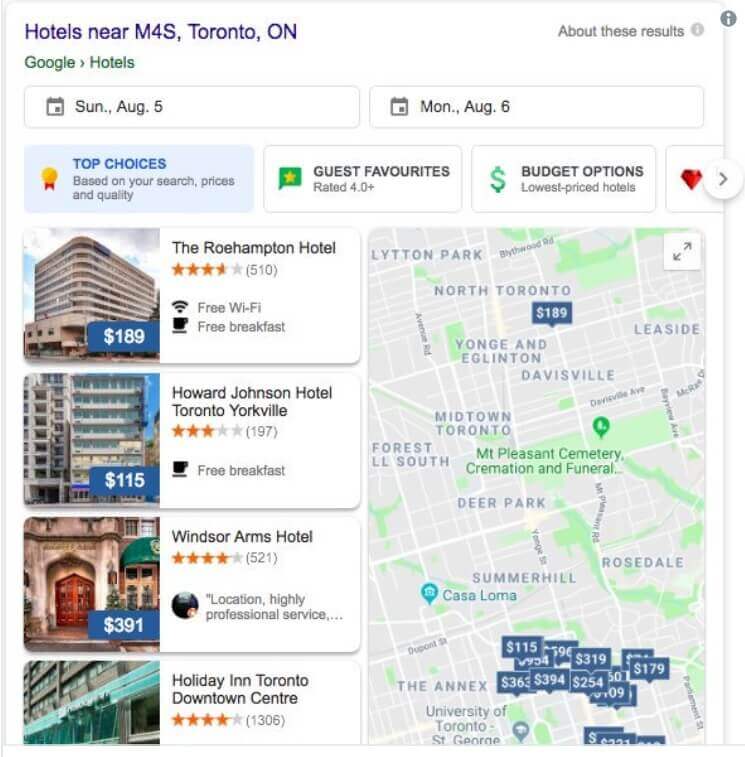This screenshot, seemingly captured from a mobile device, displays a webpage where someone is actively searching for hotels in the M4S, Toronto, Ontario area. The search query, highlighted in a purplish-blue font, is prominently positioned at the top. In the upper right-hand corner, a gray circle with a white eye icon accompanies the text "About these results."

Just below the search query, the word "Google" is displayed next to a right-facing arrow, followed by "hotels" in green text. There are two sort feature boxes at the top, each with a calendar icon: the left box shows "Sunday, August 5th," and the right box shows "Monday, August 6th," indicating the dates of the planned stay.

Below the date selectors, three categories are presented:
1. **Top Choices** (blue, with a bold blue award ribbon icon)
2. **Guest Favorites** (green speech bubble with a star icon)
3. **Budget Options** (green dollar sign icon and a red diamond-shaped gemstone)

Under these categories, four hotel options appear on the left-hand side:
1. **The Roehampton Hotel**
2. **Howard Johnson Hotel** (noted as the least expensive with three stars)
3. **Windsor Arms Hotel**
4. **Holiday Inn Toronto Downtown Centre**

Aside from the Howard Johnson Hotel, which has three stars, the other listed hotels have approximately four-star ratings. 

On the right-hand side of the page, a detailed map of the neighborhood is displayed, showing clear street names, town area sections, and neighborhood names. Towards the bottom of this map, numerous rectangular blue tags with white price points indicate the many available hotels in the area.